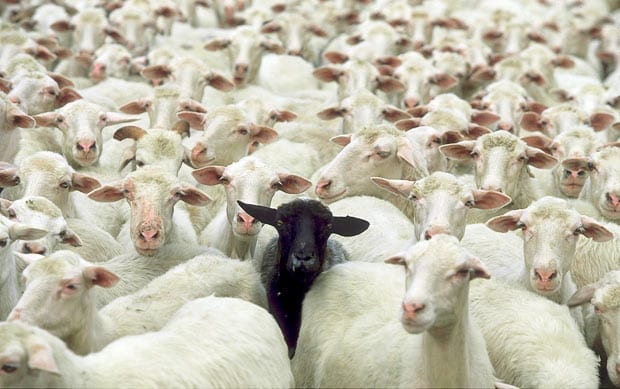The image depicts a densely packed herd of goats, primarily white or off-white in color with distinctive pink noses and pink insides of their ears. Their faces, marked by two large nostril slits, black eyes, and occasionally pink markings extending between their eyes, fill the frame from the front to the blurry background. The goats are mostly facing the camera, with their mouths closed, creating a uniform and slightly chaotic appearance. Right in the center of this cluster, a single black goat stands out, its ears jutting outward. It gazes directly at the viewer with yellow eyes, making it the focal point of the image. The photograph, taken outdoors, doesn't reveal the ground or sky, highlighting the concentration of goats. The wool of the goats appears unclean, with grey mottles visible on some. The scene is so tightly packed that only the upper bodies of most goats are visible, except for one white goat in the back middle with its mouth open, seemingly less surrounded by others and appearing a bit more isolated.